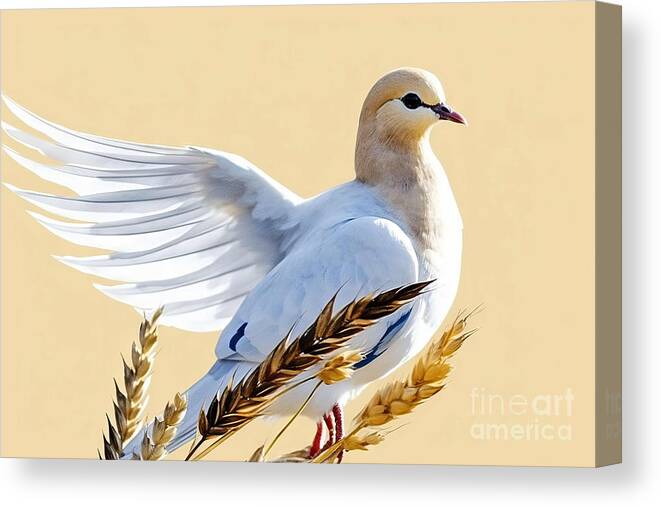This is an exquisite landscape-oriented painting of a white dove with a yellowish-brown head and a reddish beak, featuring a distinctive black stripe running from its eye to its beak. The dove is perched delicately on top of grain heads, predominantly resembling wheat, with varying shades from black and brown to golden hues. Its left wing is partially extended, showcasing its beautiful white feathers, with a touch of blue along the edge of one wing, while the right wing remains folded. The bird’s thin, red legs are visible, contributing to its elegant stance. The background of the painting is a creamy beige, giving a warm, natural feel. The artwork is presented on a slightly visible three-dimensional canvas. In the bottom right-hand corner, "Fine Art America" is subtly inscribed in a delicate white watermark.